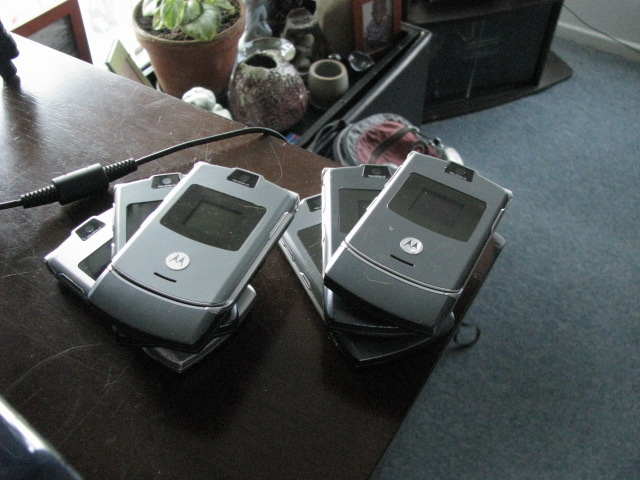In the color photo, a scene of organized clutter appears. Centered on a well-worn brown wooden table are two neatly splayed stacks of three silver-gray Motorola Razr flip phones, each featuring a black square around its front display. Dangling from the edge of the table is a conspicuous black cord, though its source remains outside the frame. The floor is covered in a grayish-blue carpet, adding a muted backdrop to the setup.

The scene extends beyond the table; in the upper portion, a pot with a reddish-orange ceramic finish houses a lush green plant. To the left, a corner of a black TV stand with glass shelving is visible, perhaps used for storing media. A smaller table or desk nearby holds a picture frame showcasing a young boy, additional plant pots, small jars, and some crystal-like formations. Against this desk leans a small backpack, complementing the scattered yet homey environment.

This detailed composition merges modern vintage technology with personal touches, creating a vivid snapshot of a past era within a lived-in space.